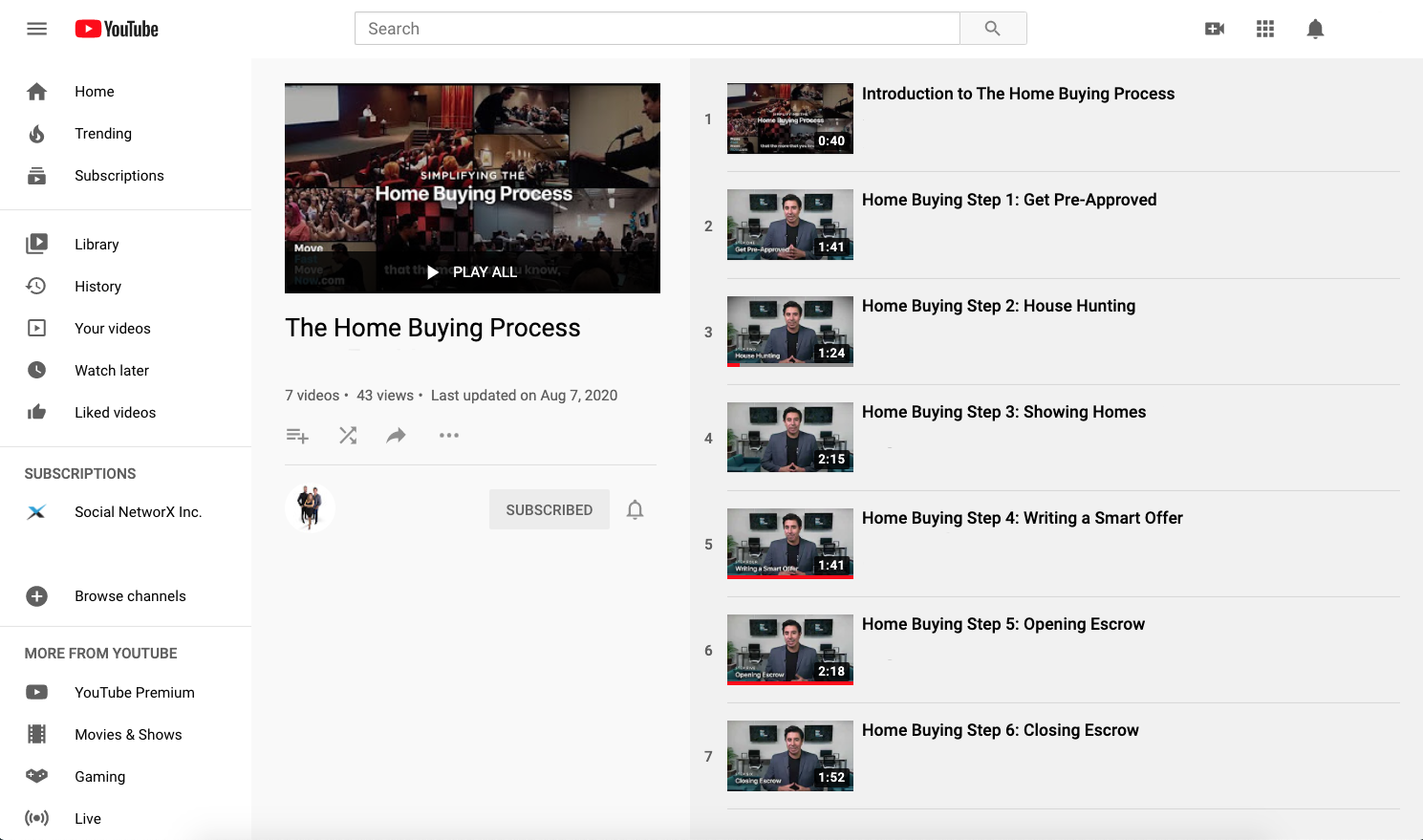This image is a detailed screenshot from YouTube featuring a white background with the YouTube logo located in the upper left corner. The logo consists of the word "YouTube" in black font, accompanied by a red square with rounded corners housing a white triangle pointing to the right. Below the logo is a gray-font sidebar listing navigation options vertically: Home, Trending, Subscriptions, Library, History, Your Videos, Watch Later, Liked Videos, and Subscriptions, followed by additional options.

The central part of the image showcases a YouTube playlist. On the left side of the playlist's section, there is a thumbnail overlaid with white text reading, "Simplifying the Home Buying Process." Directly beneath it, in white font, is the "Play All" button. Against the playlist's white background are details about the playlist: "The Home Buying Process," containing seven videos, with 43 views, and last updated on August 7th, 2020.

On the right side of this section, all seven videos in the playlist are listed vertically, each with its respective thumbnail. The titles of the videos in the sequence are: 

1. Introduction to the Home Buying Process
2. Home Buying Step One: Get Approved
3. Home Buying Step Two: House Hunting
4. Home Buying Step Three: Showing Homes
5. Home Buying Step Four: Writing a Smart Offer
6. Home Buying Step Five: Opening Escrow
7. Home Buying Step Six: Closing Escrow